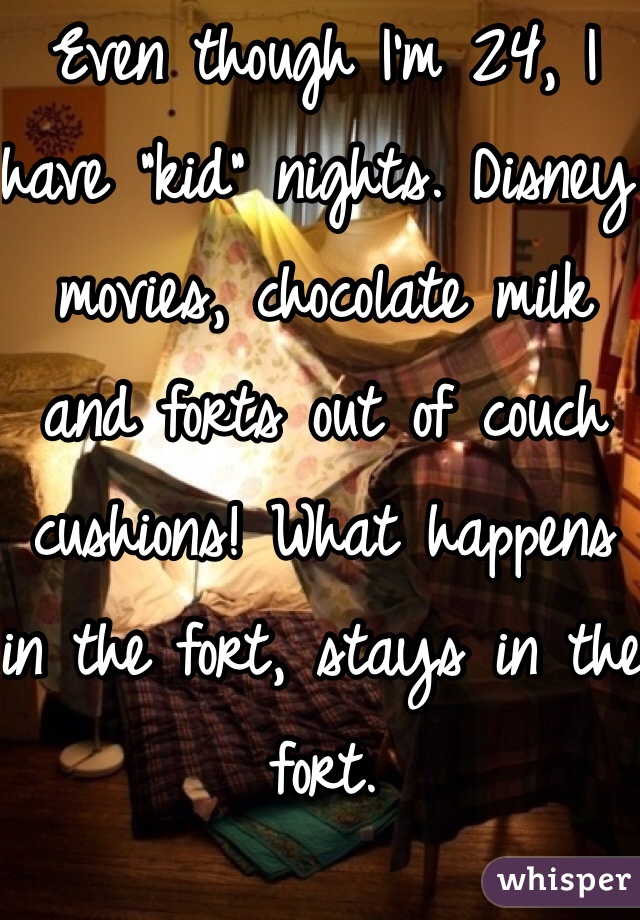The image depicts a cozy, dimly-lit living room transformed into a whimsical fort made of various cushions and blankets, showcasing a sense of playful nostalgia. Prominently displayed in white cursive text across the photo, it reads: "Even though I'm 24, I have kid nights, Disney movies, chocolate milk, and forts out of couch cushions. What happens in the fort stays in the fort." The background includes a hardwood floor, beige walls, a window with curtains, and some artwork on the walls. The scene exudes a warm, brown and beige color palette, complemented by accents of pink, green, and different shades of brown. The phrase "Whisper" is highlighted in purple in the lower right corner, indicating the source platform. The overall vibe suggests a carefree, nostalgic meme intended to be shared on social media.